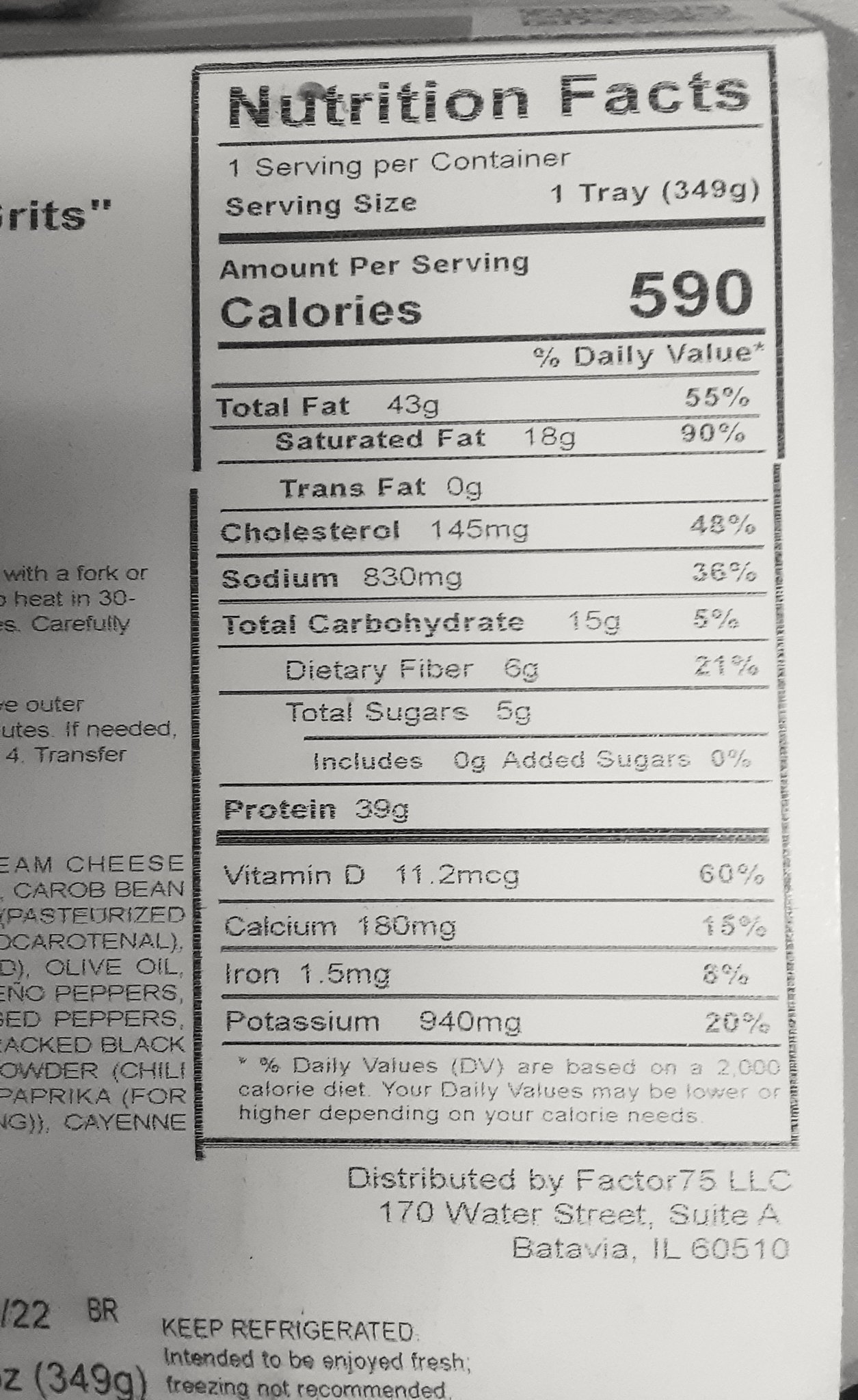This photograph shows a nutrition label on the back of a ready meal box. The label is printed on a white background with black text inside a black-bordered rectangular box, prominently displaying the heading "Nutrition Facts." The serving size is one tray, weighing 349 grams, with one serving per container. The calorie content per serving is 590. Detailed nutritional information includes total fat of 43 grams (55% DV) with 18 grams of saturated fat (90% DV) and no trans fats, 145 milligrams of cholesterol (48% DV), 830 milligrams of sodium (36% DV), 15 grams of total carbohydrates (5% DV) with 6 grams of dietary fiber (21% DV) and 5 grams of total sugars with no added sugars, and 39 grams of protein. The meal also contains 11.2 micrograms of vitamin D, 180 milligrams of calcium, 1.5 milligrams of iron, and 940 milligrams of potassium. Additionally, the label indicates that the meal is distributed by Factor 75 LLC, located at 170 Water Street, Suite A, Chavia, Illinois, 60510, and it should be kept refrigerated and enjoyed fresh. The visible part of the ingredients on the left side includes cheese, carob bean, pasteurized, olive oil, peppers, black powder, and paprika, suggesting a high-fat content dish.